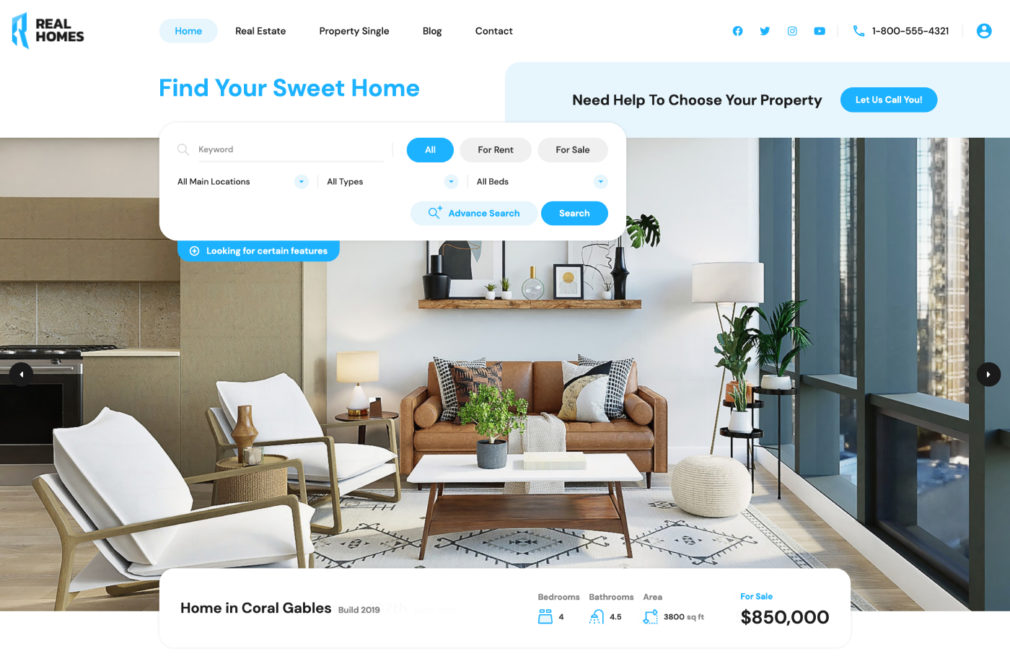The image is a screenshot from the Real Homes website, showcasing various features aimed at prospective homebuyers or renters. The interface features a prominent top navigation bar with options including "Home," "Real Estate," "Property Single," "Blog," and "Contact." Social media icons for popular platforms like Twitter, Facebook, YouTube, and Instagram are also visible, along with a contact telephone number and an account login icon.

Currently, the "Home" option is selected, triggering a search screen with the headline "Find Your Sweet Home." Users can input keywords and choose between renting or buying properties. The search functionality allows the selection of specific locations, property types, and the number of bedrooms. Both basic and advanced search options are available, with the basic search currently displayed.

In the background, there's an image of a modern designer apartment, highlighting one of the properties listed on the website. The property is for sale at $850,000, featuring four bedrooms, 3,800 square feet, and located in Coral Gables.